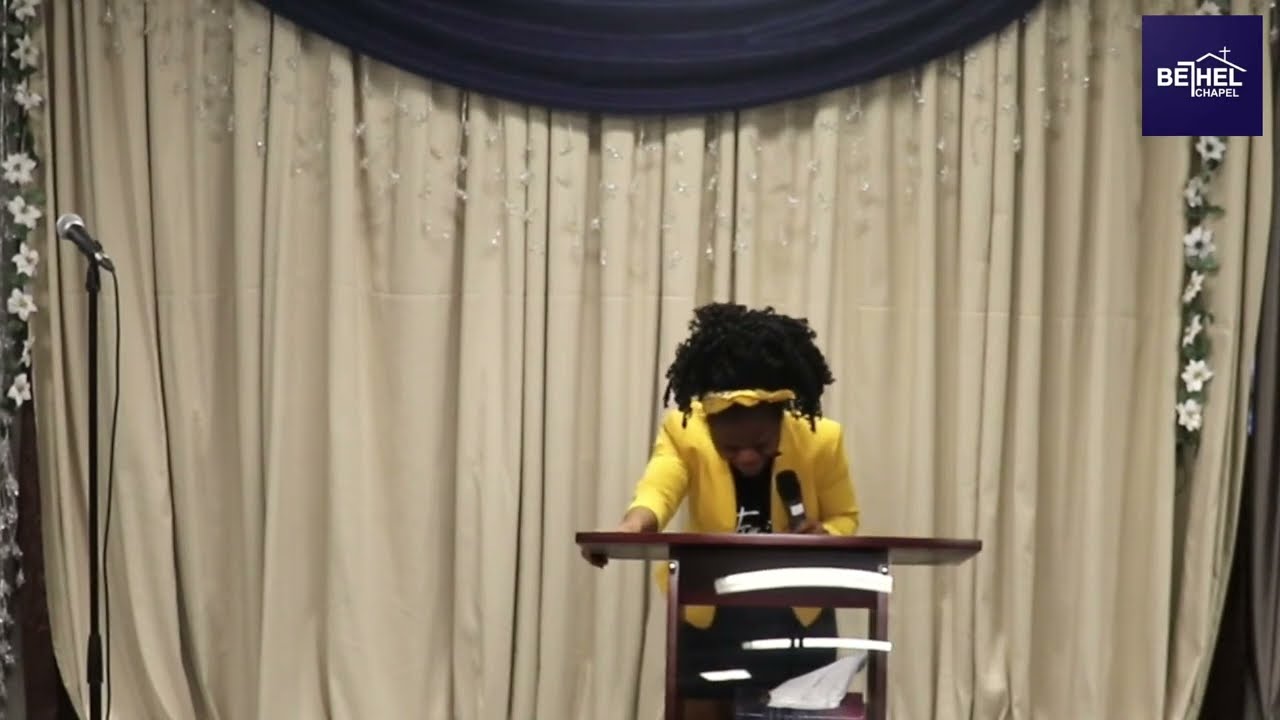A young African woman stands behind a wooden podium, holding a microphone in her left hand and leaning slightly forward, grasping the podium with her right hand. She wears a vibrant yellow suit coat over a black shirt and has a bright yellow headband securing her pulled-back short black curly hair. The backdrop features a large beige curtain with a blue awning at the top, alongside a string of white flowers adorning both sides. To her left, there is a microphone on a stand. In the top right-hand corner of the image, there is a logo that reads "Bethel Chapel" in white letters against a purple background. The setting appears to be within a church, exuding a formal and decorated ambiance.